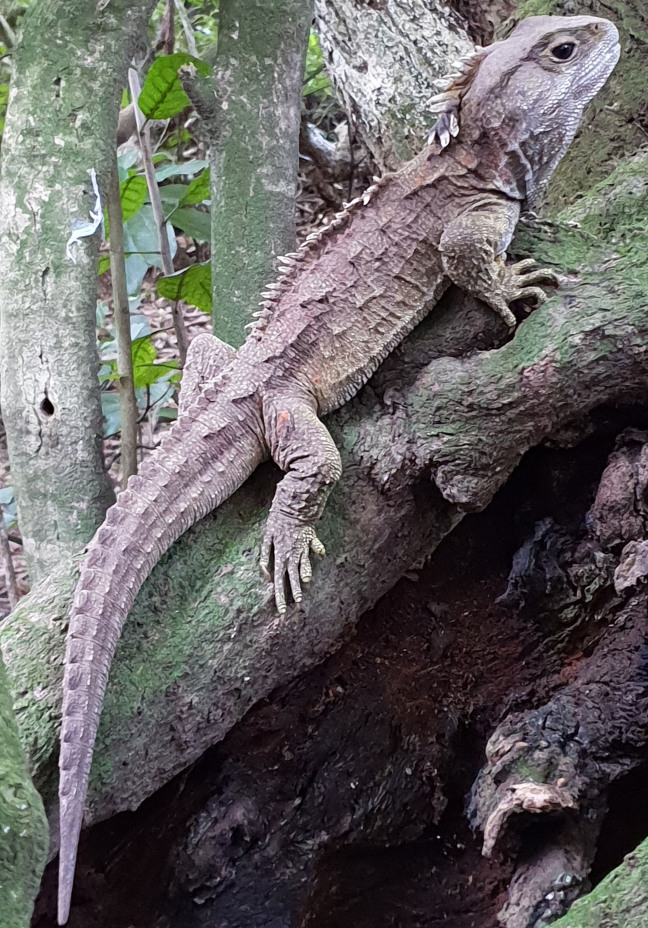In this detailed image, we see a large, brown iguana with a long, scaly tail and prominent spiky projections along its back. The iguana is gripping and climbing a slanting tree trunk, which angles from the bottom left to the top right of the photo. The tree itself is a blend of brown and green, with green moss on its surface, indicating a natural, moist habitat. The iguana's head is positioned towards the upper right of the image, while its tail stretches down towards the lower left. Surrounding the main scene, there are additional tree branches and leaves, adding abundant green hues to the overall setting, complemented by some brown tones from other tree parts and a small hole beneath the trunk. The vertical rectangular image captures the iguana in a dynamic pose, highlighting its considerable length, suggesting it might be around 18 inches.